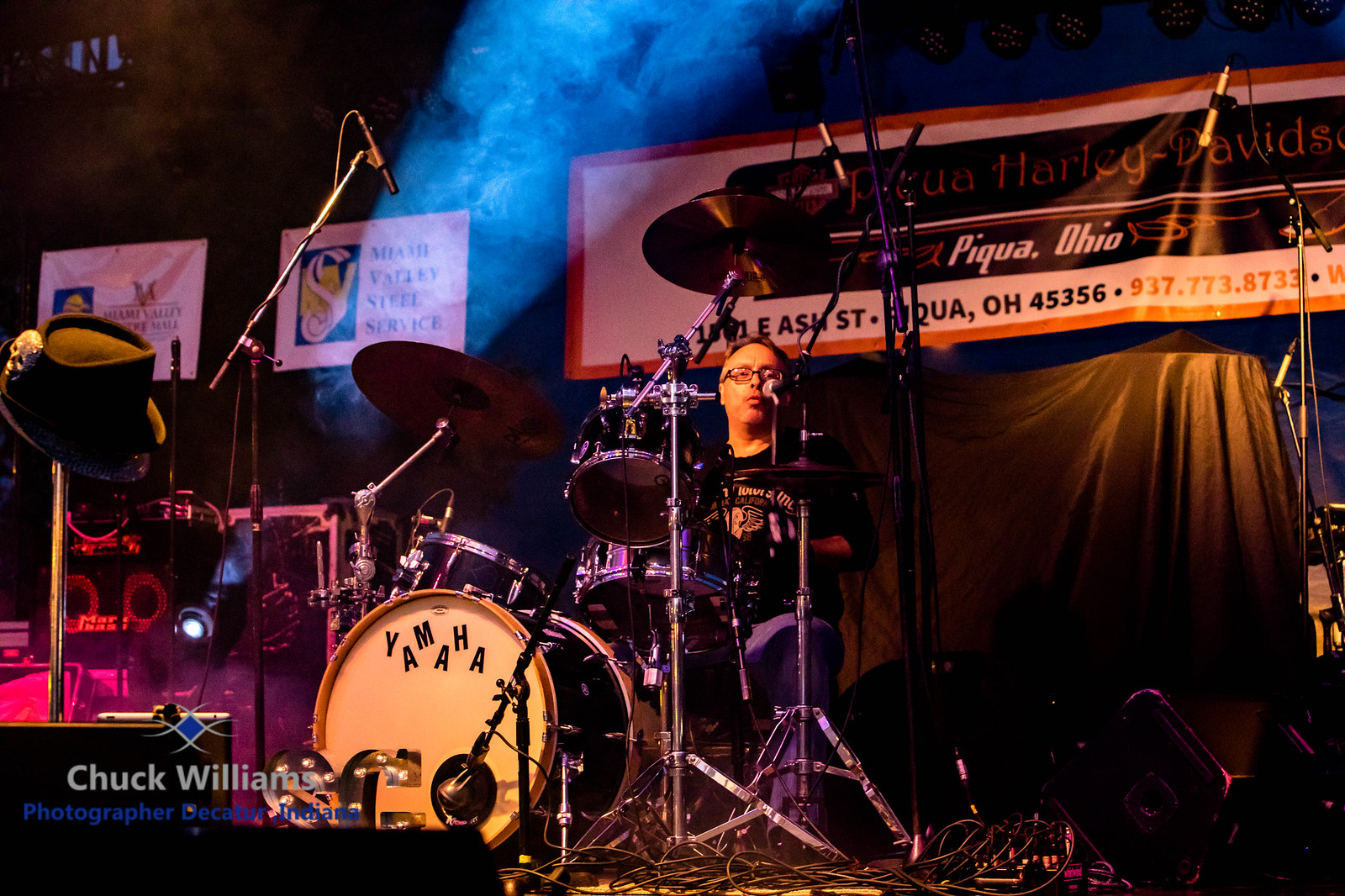The photograph portrays a drummer immersed in a musical performance, situated on a dimly lit stage. The backdrop is shrouded in darkness, punctuated by a spotlight that cuts through what appears to be a smoky or foggy atmosphere, enveloping the scene in blue hues. The drummer, wearing glasses and a black t-shirt, is captured mid-action, engaging with a microphone positioned in front of his face, suggesting he is either singing or speaking. His drum set prominently features a Yamaha kick drum with a distinctive logo of alternating letters. The stage is adorned with various equipment, including microphone stands on either side of the drummer, one of which intriguingly holds a top hat. Behind the drummer, a black tarp serves as an advertising space, bearing a banner for a Harley-Davidson dealership in Pico, Ohio. In the lower left corner of the rectangular photo, the credit reads "Chuck Williams, photographer, Decatur, Indiana."